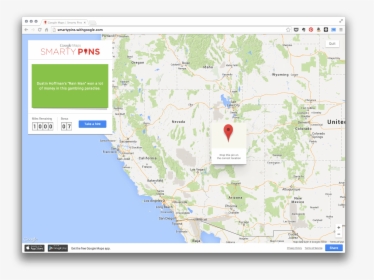A digital map displayed in a web browser dominates the image, presenting a faint and unclear view due to poor image quality. The text "Smarty Pants, Nevada, Wyoming, United States, New Mexico" is discernible, scattered across the map. States are vaguely outlined but remain largely indecipherable. The map is a mosaic of colors, including green, blue, white, and red. Two distinct markers are visible near the center: one red and one blue, perhaps denoting specific locations or points of interest.